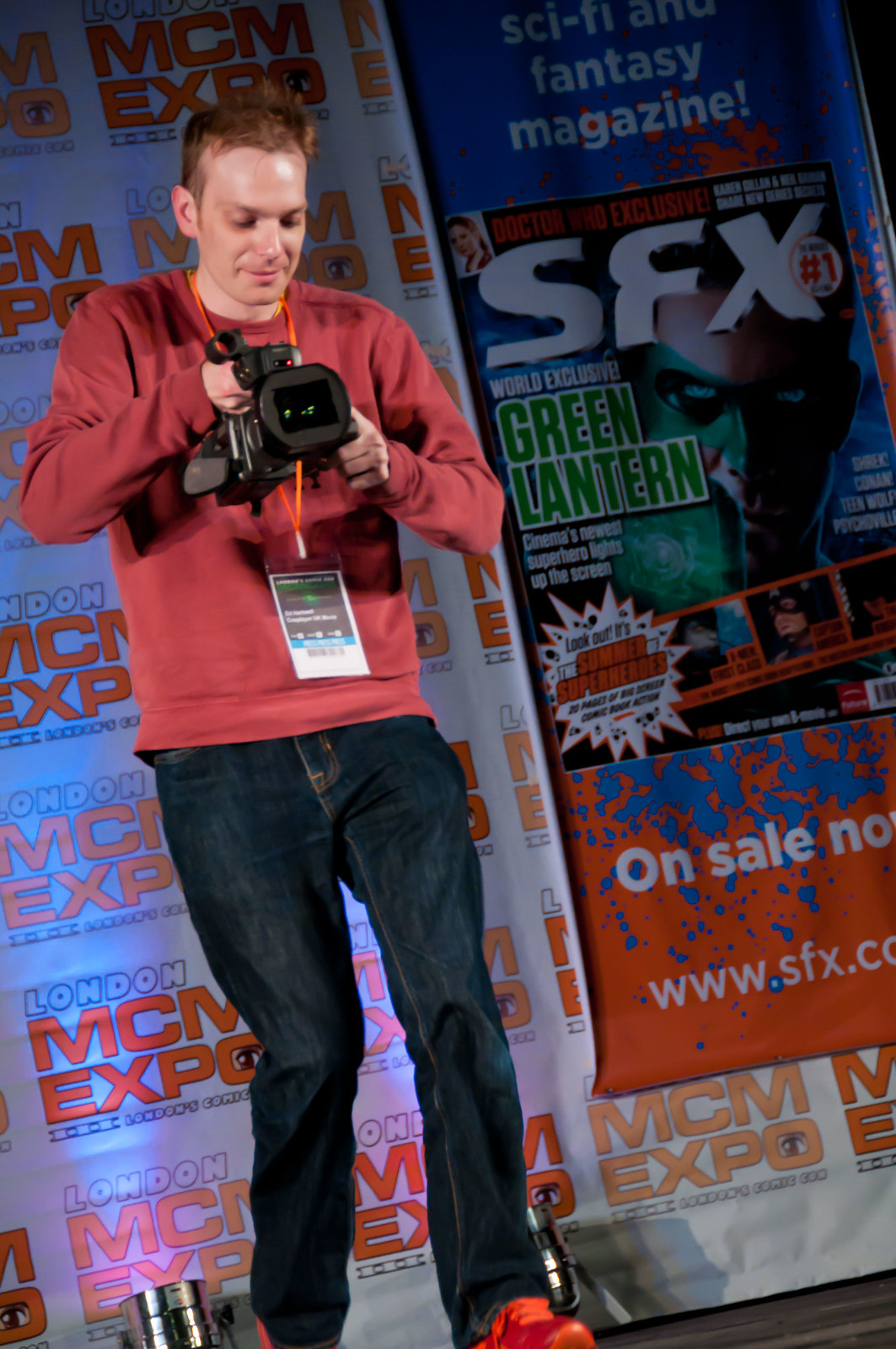This vertical indoor photograph captures a man standing on a stage, tilted slightly to the left. The man, of Caucasian descent with short, reddish hair, is wearing a long-sleeve red sweater, baggy dark blue jeans, and red tennis shoes. He is intently looking down at the screen of the video camera he holds with both hands. Around his neck hangs a red lanyard with a white pass attached. Behind him, the banner on the left reads "London MCM Expo" in white with a blue outline, and "MCM Expo" in orange. To his right, another banner advertises "Sci-Fi Fantasy Magazine," featuring a cover image of Ryan Reynolds as Green Lantern, with text proclaiming "On Sale Now" and the website "www.sfx.com." The stage is lit by two spotlights pointing upwards, enhancing the clarity of the banners at the back.